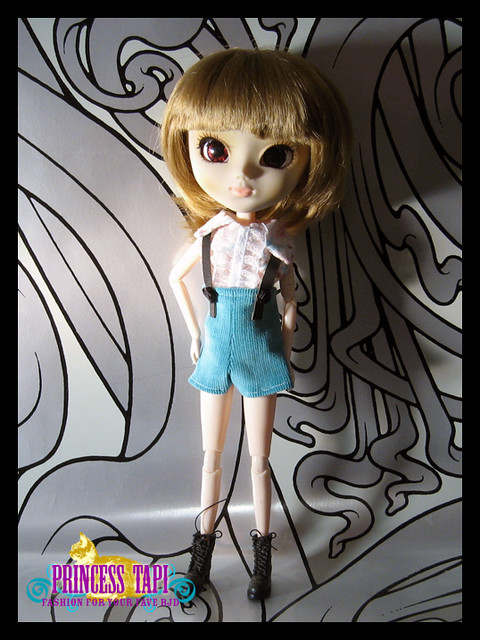The image features a highly detailed, stylish doll that exudes youthful charm. She stands confidently in front of a swirling gray and white backdrop reminiscent of spaghetti lines. The doll has short brown hair styled in a neat bob with straight-cut bangs. Her facial features are incredibly expressive, with large brown eyes framed by long eyelashes and accentuated by red-brown eyes. Her lips are subtly colored with a beige lipstick, enhancing her mature, yet youthful appearance, suggestive of an Asian heritage. 

She is dressed in a short-sleeved white buttoned shirt with a collar, paired with blue jean shorts held up by suspenders, creating a modern, playful look. The ensemble is completed with high lace-up black boots that extend above her ankles and showcase her long, thin legs. The lighting accentuates her features, casting a soft glow on her left side while leaving the right side slightly shadowed, adding depth to her appearance.

To the left bottom of the backdrop, the image prominently displays the text "Princess Tappy" in purple, followed by "Fashion for your fave BJD," confirming the doll as a Ball-Jointed Doll (BJD). The overall composition and outfit suggest a character that bridges the gap between fashion-forward and youthful innocence, likely appealing to a teenage or young adult audience.